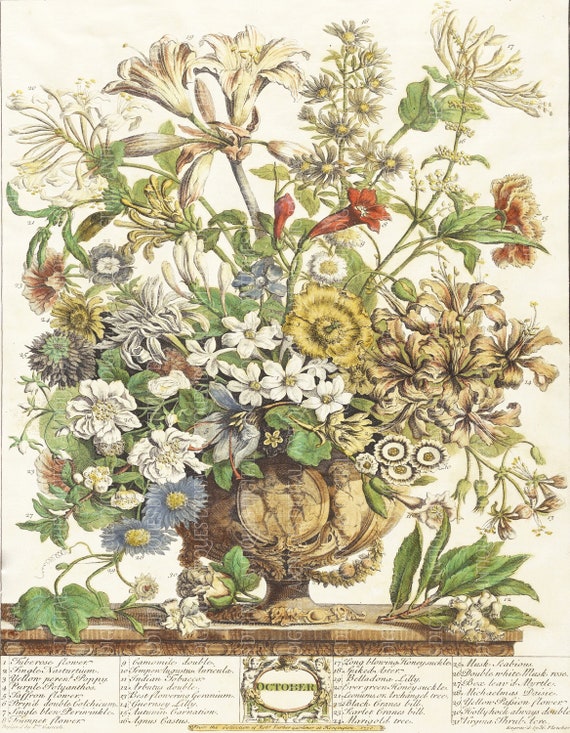This classical illustration, reminiscent of the 1800s and possibly created using a lithograph style that originated from a pencil sketch, showcases a diverse bouquet of flowers arranged in a highly detailed, pedestal-like urn or goblet-shaped container. The tan-colored vase or urn sits on a table, its flowers splaying out in all directions, embodying a Victorian aesthetic. The bouquet includes a variety of colored flowers, such as blue daisies, white lilies, tiger lilies (orange-flowered variety), pink blossoms, black-eyed Susans, and what appear to be blue orchids with sunflower-like patterns. The illustration features some fallen flowers and leaves on the table surface below the vase, adding to the natural charm of the scene. The leaves are vividly green, enhancing the muted yet diverse color palette of the bouquet. Notably, the word "OCTOBER" is inscribed in small, capitalized font beneath the flowers, surrounded by an oval filigree decoration. This text, alongside possible numbered flower descriptions, suggests that the illustrated blooms are characteristic of October.